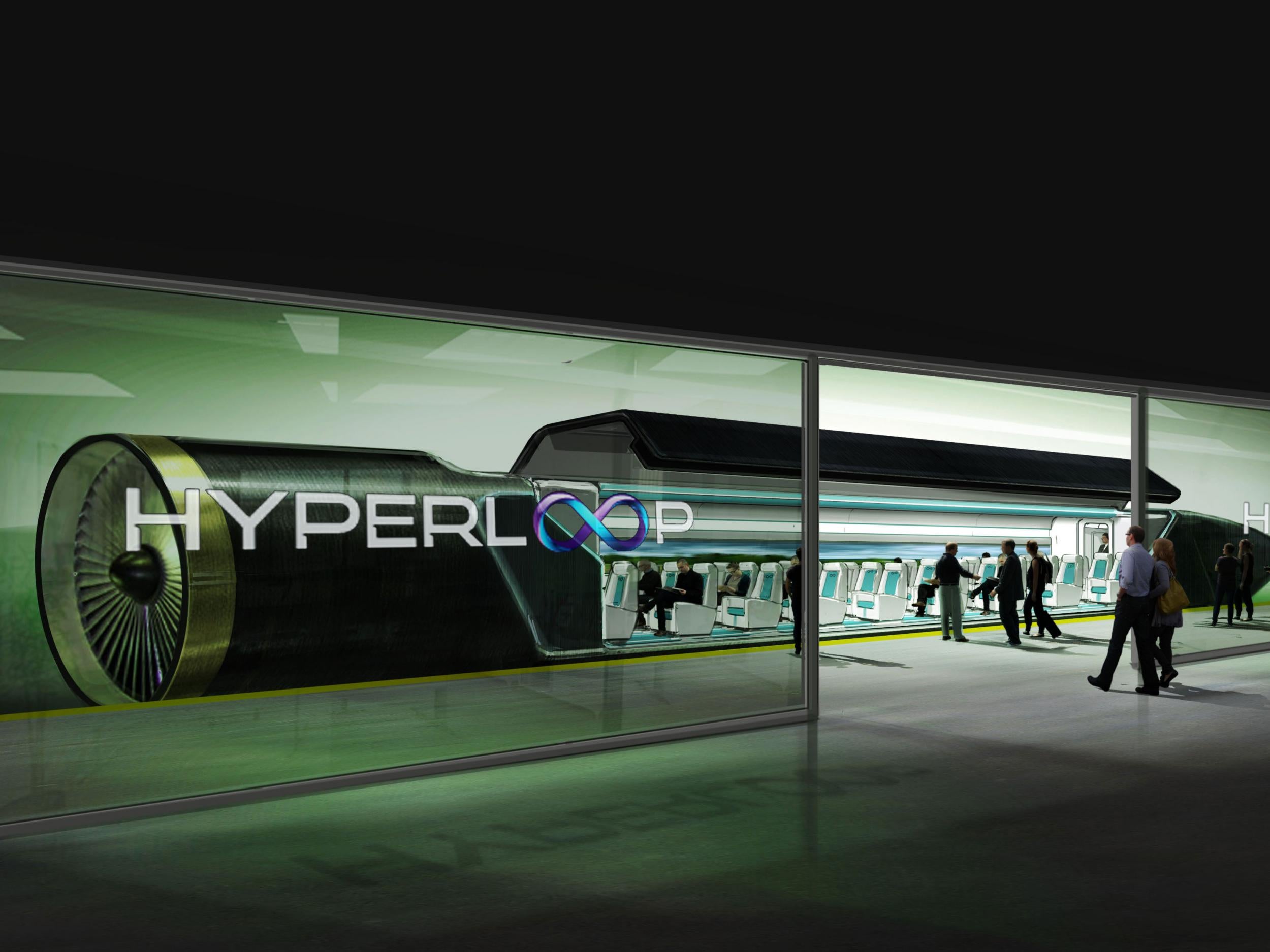The image is an artist's digital rendering of a futuristic Hyperloop high-speed mass transit system. This indoor scene showcases a sleek, almost bullet-shaped transportation vehicle, which is designed to revolutionize the way we travel by achieving speeds of 200 to 300 miles per hour. The upper third of the image is predominantly black, highlighting the central elements below. Dominating the scene is a cylindrical black Hyperloop pod with a distinctive design—a narrow front tapering to a more circular rear featuring a large, black conical fan with silver flat blades.

The Hyperloop pod is situated behind slightly tinted glass windows, adorned with the word "Hyperloop" in large, white bold letters, and the 'OO' of 'loop' creatively represented by a purple and blue infinity symbol. The glass panel also has an opening that allows passengers to board. The Hyperloop's side door, which opens upwards, reveals a row of white and light blue seats, some occupied by seated passengers, while others are entering the tube. The ground beneath this entire setup is grey, enhancing the contrast and making the sleek, futuristic design stand out even more. Several people can be seen walking through the doorway, highlighting the realistic interaction with this next-generation high-speed rail system.